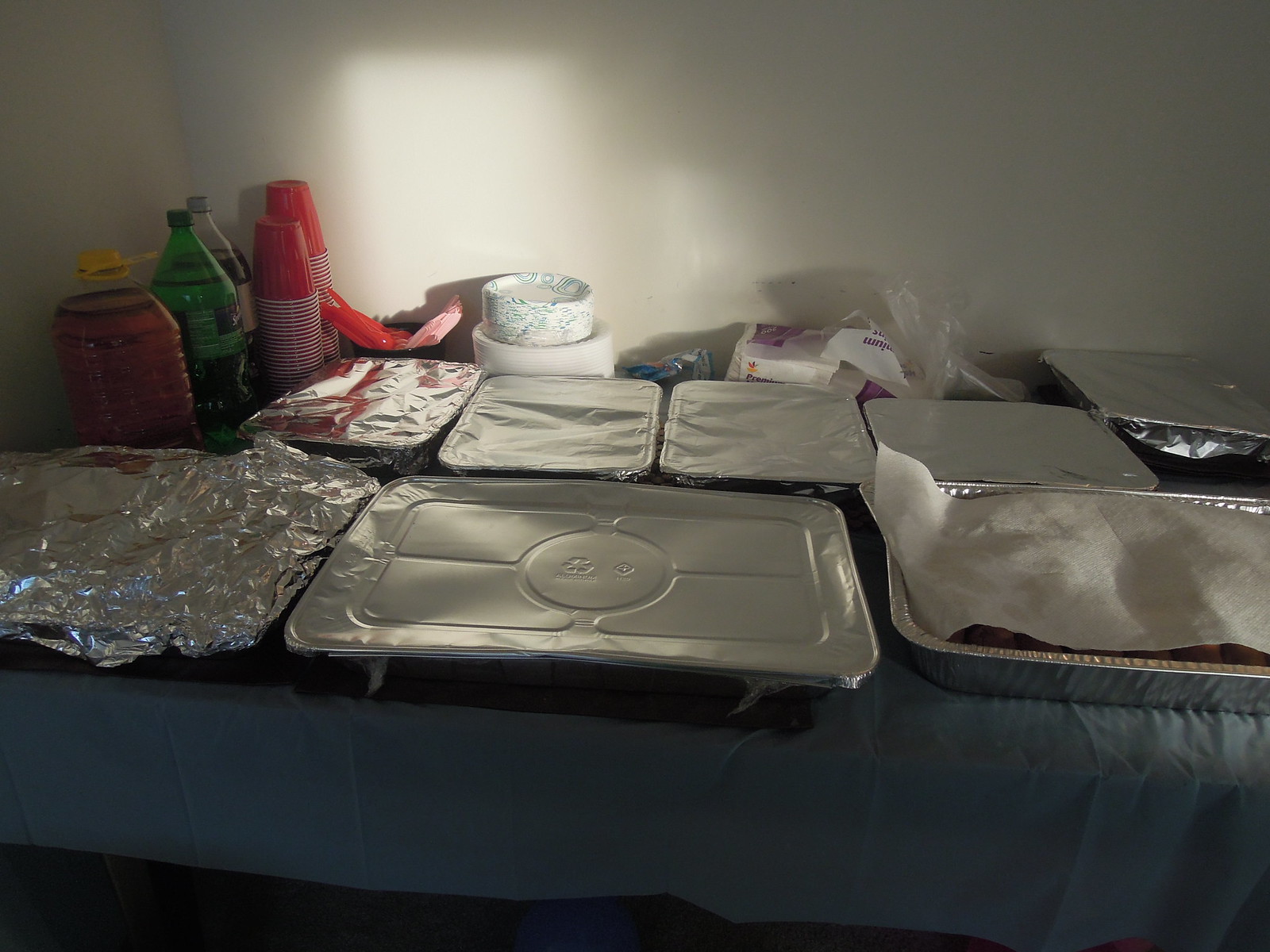This image captures the early setup of a dinner party or potluck, characterized by a darkly lit room with a light gray wall in the background. A long table draped in a thin blue plastic tablecloth stretches out, laden with preparations for the event. Dominating the table are several large, disposable aluminum food trays, mostly covered, hinting at the awaiting feast. One particularly stands out with a paper towel laid on top instead of a lid. On the left side of the table, there are two stacks of red Solo cups, flanked by two-liter bottles of soda—one cola and one clear drink—and a jug of juice. Adjacent to these are paper plates and a potential pack of napkins or utensils, suggesting an organized setup for guests to easily serve themselves. Additionally, a box of disposable gloves can be seen in the back, ensuring hygiene. Small red decorations hang above, adding a festive touch to the scene despite the subdued lighting.